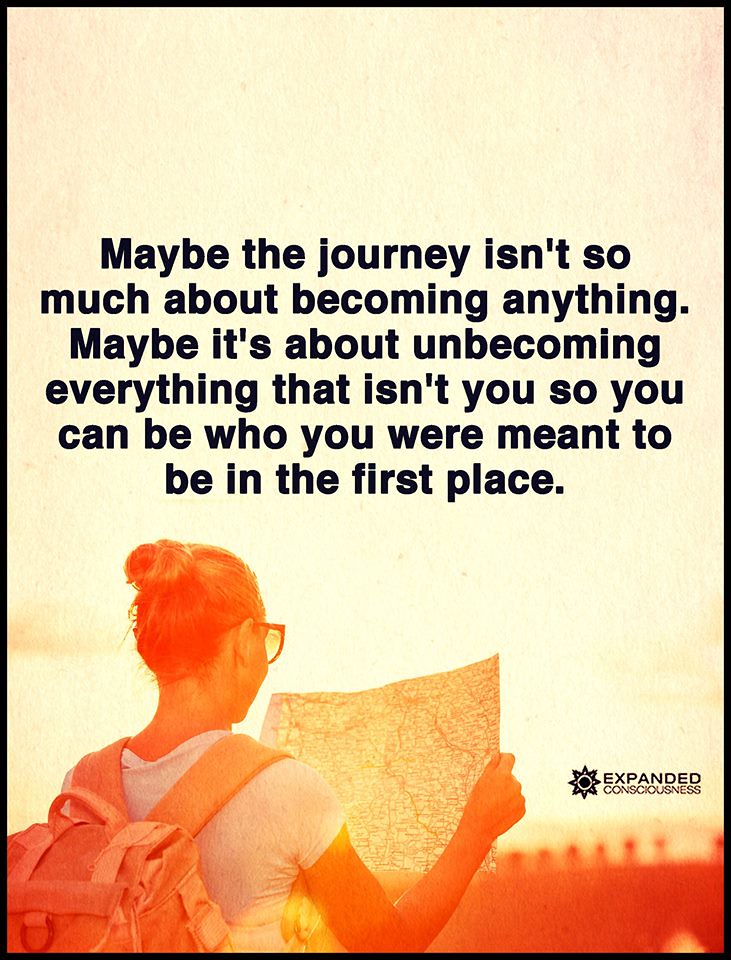The poster features an ethereal, yellow-orange background that fades from peach at the top to deep red at the bottom, casting an orangish hue over the entire image. At the forefront, a young Caucasian woman with blondish hair tied up in a bun and glasses is intently looking at a large map she holds with both hands, facing slightly away from the camera. She wears a white t-shirt and a tan backpack. The black, bold text above her reads, "Maybe the journey isn't so much about becoming anything. Maybe it's about unbecoming everything that isn't you, so you can be who you were meant to be in the first place." To the right of the map, a small star or compass logo is visible with the text "expanded consciousness" beside it. The entire scene is infused with a soft, dreamy blur that adds to the inspirational tone of the poster.